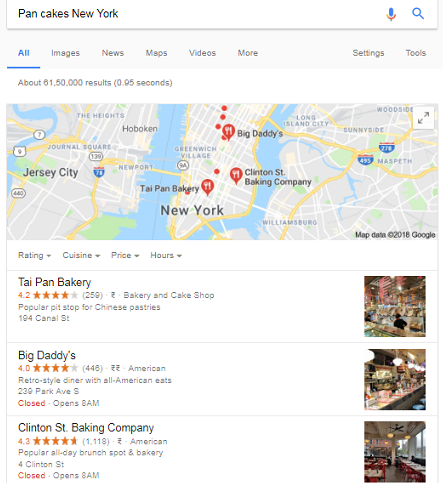The image shows a web search on a computer with the query "pancakes New York" entered into the search bar. The display includes a map centered on New York City and Jersey City, highlighting three prominent pancake locations: Big Daddy's, Clinton Street Baking Company, and Tai Pan Bakery.

1. **Big Daddy's**: An American retro-style diner with an "all-American eats" theme. Despite being currently closed, it opens at 8 a.m. The address is provided, and the diner has earned four stars based on 448 reviews. The interior dining area is also depicted in an accompanying image.

2. **Clinton Street Baking Company**: Renowned as a popular all-day brunch spot and bakery. This location boasts a rating of 4.3 stars from 1,118 reviews. Similar to Big Daddy's, it is currently closed but will open at 8 a.m. The image included shows the bakery's interior dining space.

3. **Tai Pan Bakery**: Known for its bakery and cake shop offerings, with a specialization in Chinese pastries, making it a popular pit stop. It has garnered a rating of 4.2 stars out of five from 250 reviews. The bakery is located at 194 Canal Street, and its exterior can be seen in the included image.

Each bakery description provides valuable details such as star ratings, reviews, popular offerings, operating hours, and images, aiding in the selection of a pancake destination in New York City.